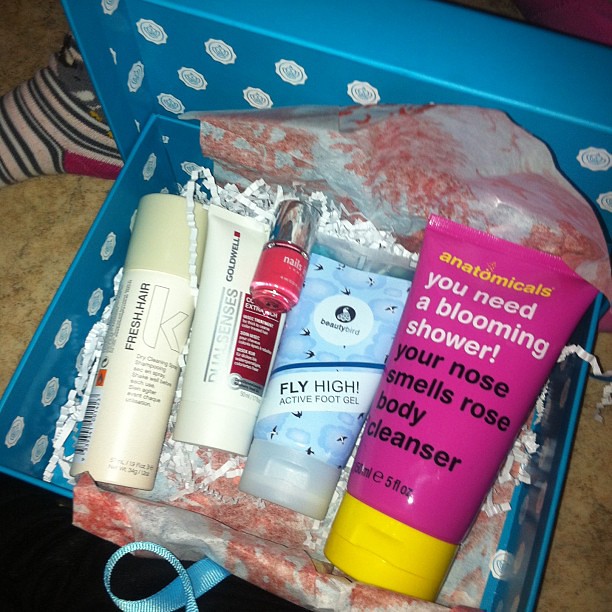The image depicts a meticulously arranged gift box filled with various beauty and personal care products. The box itself is bright blue, adorned with white circular floral patterns and lined with red and white tissue paper, along with shredded filler material to enhance its presentation. The box appears to be placed on a countertop, with its lid resting nearby.

Inside the box, several bottles and containers are neatly arranged. On the left, there is a light beige spray can labeled "Fresh Hair," featuring a large 'K' on its design. Adjacent to it is a white squeeze tube of "Dual Senses Goldwell." Next is a small, silver-capped bottle containing red nail polish, which has 'nails' inscribed in white letters. Moving further to the right, there's another tube with cute blue cartoon chicks design, labeled "Beauty Bird Fly High Active Foot Gel." Finally, on the far right, a bright purple squeeze bottle with a yellow cap stands out, labeled "Anatomicals You Need a Blooming Shower Your Nose Smells Rose Body Cleanser" in playful fonts, holding 150 milliliters (5 fluid ounces) of product.

At the very upper left of the image, one can glimpse the heel and arch of someone's foot adorned in a stripy sock, adding a touch of casual human presence to the well-curated display of hygiene and beauty products.